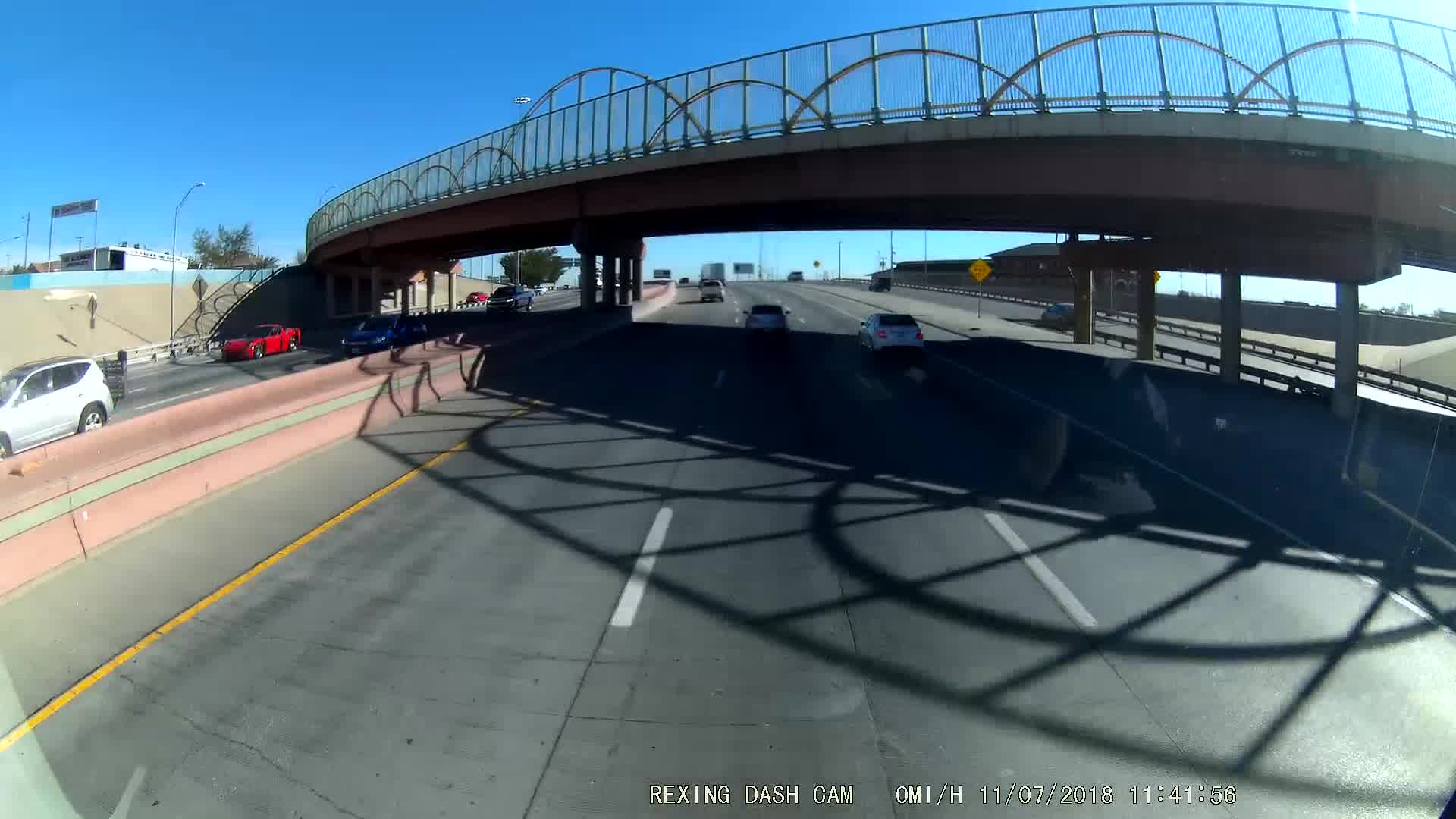A high-resolution photograph captures a visually striking bridge spanning an expressway. The bridge, with its artistic design, features a series of arches of varying heights along its fence line, giving it an elegant and modern appearance. Imprinted at the bottom of the image are the details "Rexine dash cam, O-M-C-M-L/H, 11-1-2018, 11:41:56," suggesting the photo was likely taken by a truck driver due to the elevated perspective of the scene. Below the bridge, a three-lane highway unfolds, with two white cars visible in shadow under the structure. The vehicles occupy the center and right lanes, with the car in the middle lane positioned approximately one car length ahead of the one in the right lane. The left-most lane remains free of traffic in this particular moment.